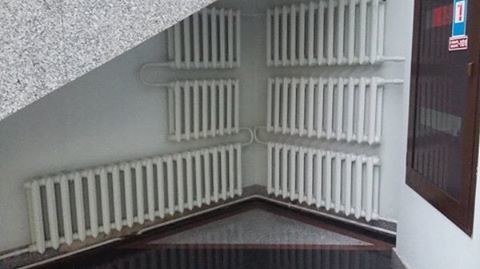This color photograph captures the corner of a room where an array of interconnected radiators is situated beneath a diagonally sloping feature that appears to be stairs. The flooring under the diagonal section features a gray and white speckled pattern, consistent with the side walls, which may be marble. The floor itself mirrors this with a similar gray and white pattern, accented with a dark brown or possibly red-bordered triangular section in the corner and a highly polished black floor extending beyond that.

The radiator setup involves six units of varying lengths. Along the left wall is a notably long radiator at the bottom, connected by pipes that form a horseshoe bend to two smaller radiators stacked directly above it. On the right wall, a similar arrangement is observed with three connected radiators: a small one which is linked to another small radiator above it, and both are in turn connected to a medium-length radiator at the top.

All the radiators are interconnected with pipes that enter from the lower left, loop through each radiator, and exit through the lower right, where they disappear behind a wall. This wall features a glass case possibly related to fire equipment; however, the label is too small to decipher thoroughly, though it appears to show a fire extinguisher symbol on a white background with a blue label, and a red label with white text beneath it.